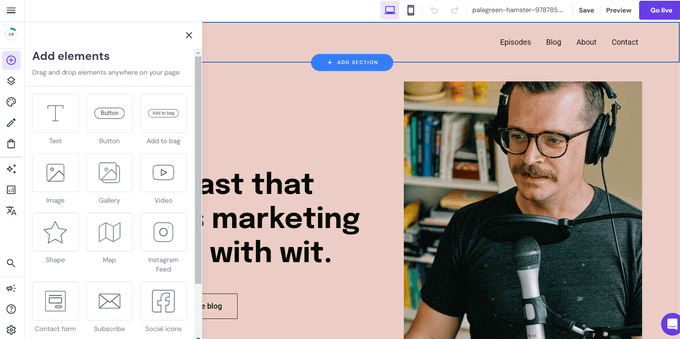Screenshot of a Website Editor Interface

In this detailed image, we see a screenshot of a website editor interface, showcasing various tools and elements available for web design. On the left side of the screen, a vertical menu bar is populated with numerous icons, each representing different functions. The highlighted icon, a circle with a plus sign in the center, stands out against a purple background, indicating it is currently active.

Upon selecting this icon, a submenu titled "Add Elements" has popped up, presenting a drag-and-drop system for incorporating elements into the web page. The options are displayed as a series of squares, each containing an icon and a label:

1. **Text**: Represented by a 'T' icon.
2. **Button**: A rounded button labeled "Button".
3. **Add to Bag**: A button labeled "Add to Bag".
4. **Image**: A square icon with a minimalist line drawing of a mountain.
5. **Gallery**: Similar to the Image icon but with an additional overlapping rectangle.
6. **Video**: Featuring an outline of the YouTube logo.
7. **Shape**: Denoted by a star icon.
8. **Map**: Illustrated with an icon resembling a folded brochure map.
9. **Instagram Feed**: Marked by the Instagram logo.
10. **Contact Form**: An icon representing a standard form.
11. **Subscribe**: Symbolized by an envelope.
12. **Social Icons**: Displaying the Facebook logo.

The website currently being edited features a background and partially visible black text obscured by the "Add Elements" menu. 

At the top right of the interface, a navigation menu offers links labeled Options, Episodes, Blog, About, and Contacts. Below this is an image of a man with glasses and a mustache, wearing black headphones and speaking into a microphone, suggesting the website might be related to a podcast.

This screenshot provides a comprehensive view of the web design tools and the layout elements ready for customization.